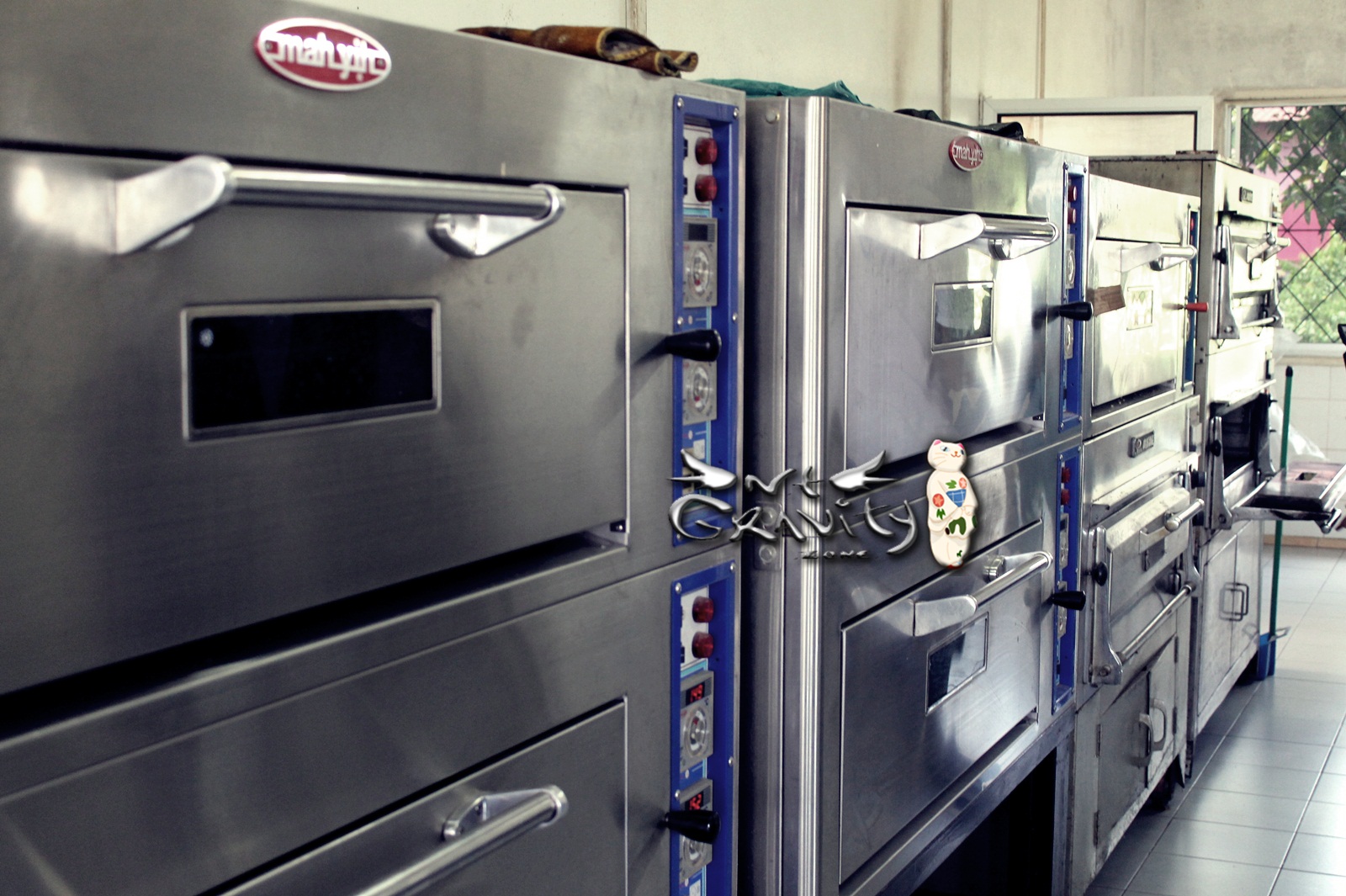The image depicts a pristine industrial kitchen, likely in a restaurant, featuring six to eight silver convection ovens aligned in a diagonal line stretching towards the back of the shot. These heavy-duty ovens, speculated to bear the brand name "Ma Y-A-I-H," are equipped with detailed control panels that feature four red knobs arranged in a square with blue bordering. On the top of the nearest ovens, there are multiple sets of silicone oven mitts in brown, turquoise blue, and black. A sign at the forefront reads "Gravely" in a stylized font, possibly indicating a product line for industrial cooking equipment.

The kitchen floor is covered in gray stone tiles, keeping with the industrial aesthetic. Sunlight pours in from a gridded window at the end of the room, providing a view of green trees outside and casting a light glow over the space. A notable detail includes one of the oven doors being open, revealing a dark interior, and a dustpan located nearby. The overall scene suggests a clean and well-organized kitchen, ready for industrious use.